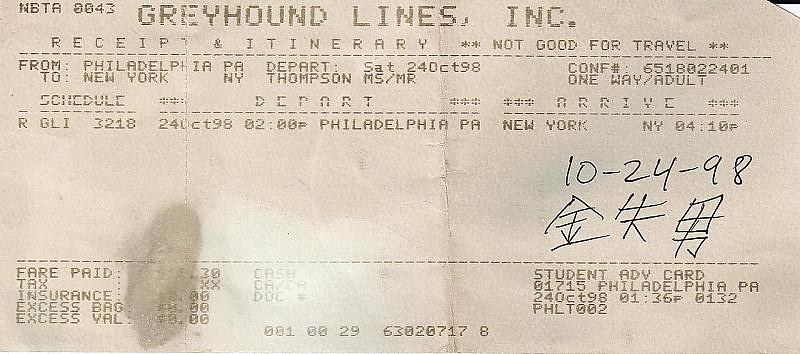This close-up photograph showcases an old, worn Greyhound bus ticket, dated 10-24-98. At the top, in light gray font, it reads "Greyhound Lines, Inc." and states "Receipt & Itinerary **NOT GOOD FOR TRAVEL**" beneath a dotted line. The ticket details a journey from Philadelphia, PA to New York, NY, departing on Saturday, October 24th, 1998. It bears a confirmation number 6518022401 and is marked as a one-way adult fare for Mr. or Mrs. Thompson. Notably, there are handwritten Chinese characters next to the date. Although much of the fare information is smudged, you can discern mentions of taxes and other fees. The ticket also references a "Student Advice Card". Additionally, a scheduled departure time of 2:00 PM from Philadelphia with an arrival in New York at 4:10 PM is indicated. The photograph highlights the worn and somewhat faded nature of the ticket, emphasizing its age and use.